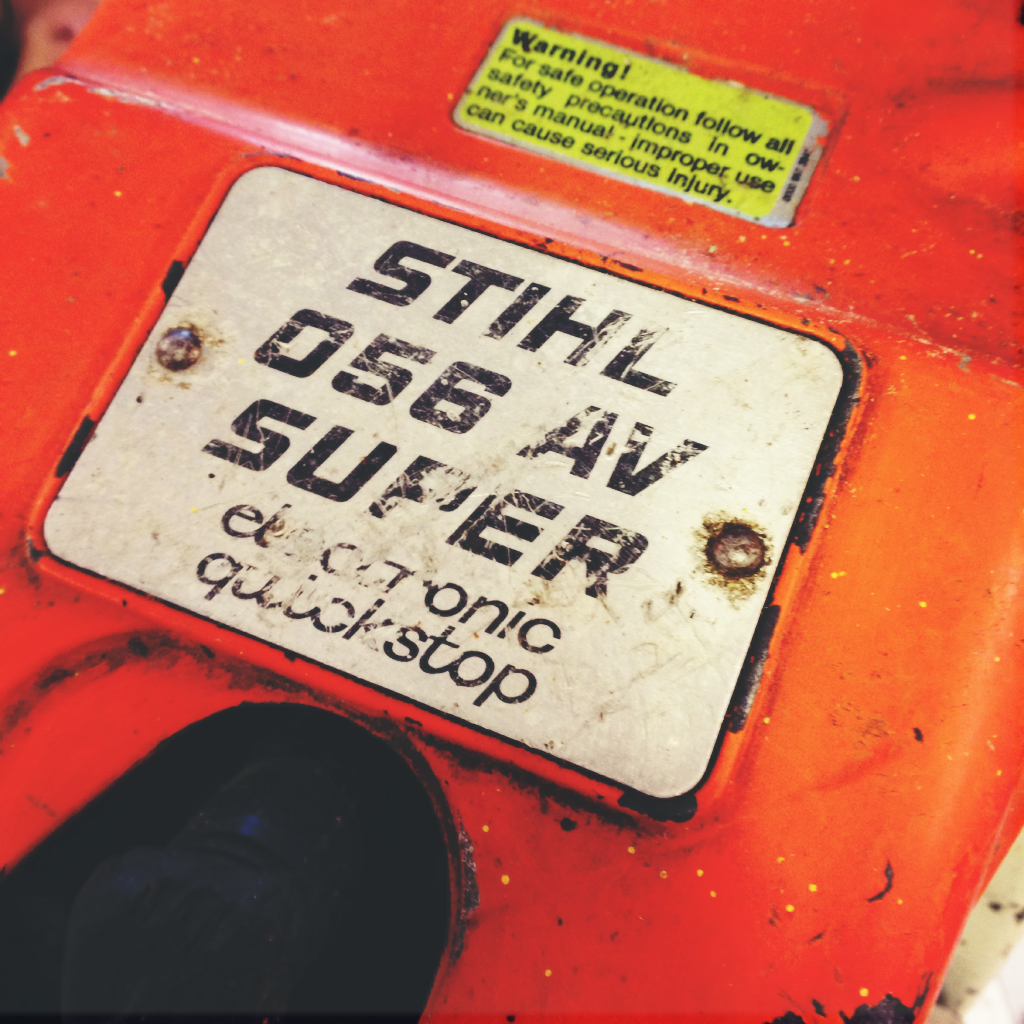This photograph features a close-up of a power tool's ownership plate, prominently labeled "Stihl 056 AV Super Electronic Quick Stop" in bold black lettering. The plate is mounted on an orange body of heavy machinery, secured with bolts. Above the plate is a neon yellow warning tag that advises, "WARNING: For safe operation follow all safety precautions in the owner's manual. Improper use can cause serious injury," also in bold black text. Additionally, a noticeable black circular component is attached to the tool's bottom left side, further indicating the complexity and industrial nature of this equipment.